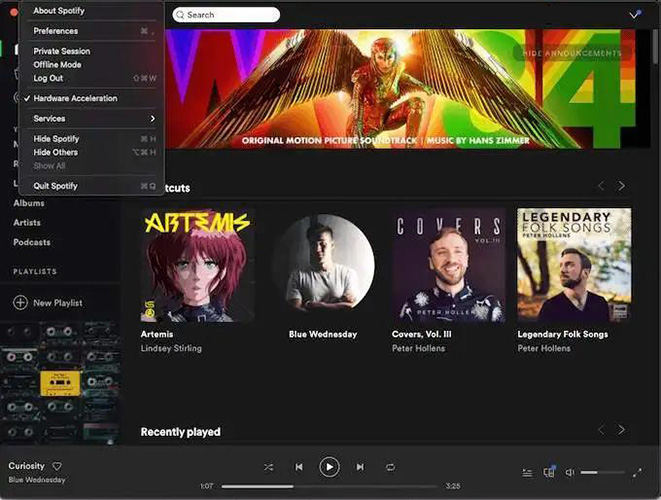This image displays a Spotify web page interface. At the top left, there's a small red circle next to the text "About Spotify." A drop-down menu is open, revealing several options: Preferences, Private Session, Online Mode, Logout, Hardware Acceleration, Services, Hide Spotify, Hide Others, Show All, and Quit Spotify. To the right of "About Spotify," there is a white oval search bar labeled "Search."

Below this, there's a striking image of a woman in a gold outfit with matching gold wings, standing against a vibrant background displaying the characters "W84." The text beneath the image reads, "Original Motion Picture Soundtrack Music by Hans Zimmer." Partially obscured by the drop-down menu is the term "TCUTS."

Further below, several icons are displayed. The first icon features an illustration labeled "Artemis," showing a red-haired woman in a black, tight outfit titled "Artemis Lindsey Sterling." Next to it, an icon shows a man standing with his arms crossed in front of a white and black wall, wearing a white t-shirt. This is titled "Blue Wednesday." Another icon nearby is for "Covers Volume 3" by Peter Hollens, showing Peter Hollens with a beard and mustache, wearing a black shirt adorned with white sparkles. On the far right is an image of a man with a mustache and beard, wearing a V-neck black shirt, titled "Legendary Folk Songs by Peter Hollens."

At the bottom of the page is a section labeled "Recently Played," and at the very bottom are the playback controls for selecting and playing songs. The currently highlighted song on the far left is "Curiosity" by Blue Wednesday.